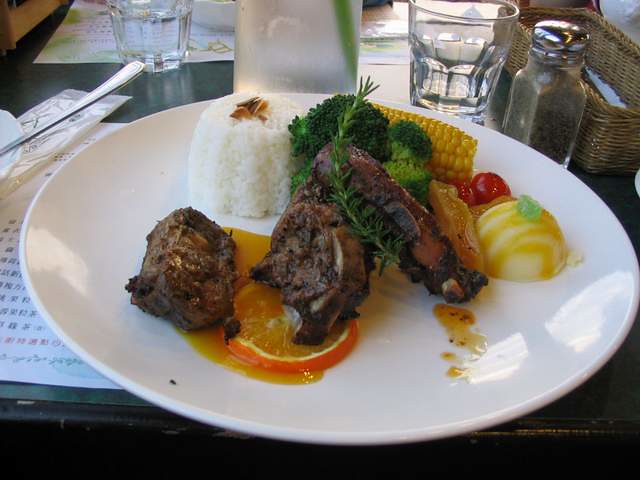The photograph shows a carefully plated meal on a white round dish, positioned centrally on a black table. The dish features two halves of heavily seared or roasted meat, possibly beef or steak, placed on the lower left side of the plate, around the 7 o'clock position. The meat rests on a slice of orange. 

To the upper right of this meat-orange combination, there is another slice of dark, roasted meat. Right above the meat on the orange slice, and slightly to the left, sits a big spoonful of white rice, which appears sticky. Adjacent to the rice, on the right, are three or four small crowns of broccoli. Just behind the broccoli and to the right is an ear of corn on the cob, and further right, there are two red cherry tomatoes. In front of the cherry tomatoes lies a yellow and white dome-shaped food item, which has a gummy appearance, though its exact nature is unclear.

The background features a clear glass and a dark brown pepper shaker with a metal cap, positioned at the top right. A light brown basket is situated behind these items. In the upper left corner, there is a partially visible piece of silverware, presumably a metal spoon, and behind it, another empty glass. The overall setting appears to be a daylight scene, possibly captured at a restaurant, focusing on a well-presented meal ready to be enjoyed.